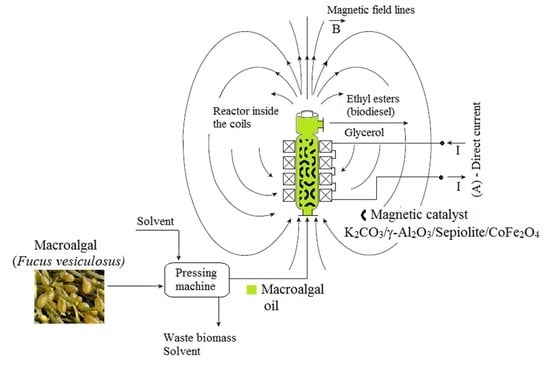The image is a detailed scientific diagram depicting a reactor setup for processing macroalgal oil into useful products. Central to the image is a green cylinder labeled "reactor," with "reactor inside the coils" noted within the diagram. Surrounding the cylinder are black boxes with Xs, likely representing magnetic catalysts involved in the reaction. Extending from the top and bottom of the cylinder, there are lines marked "magnetic field lines," indicative of the forces at play in the setup.

In the lower portion of the diagram, several terms are listed, including "micro algal solvent," "pressing machine," "waste biomass," and "solvent," indicating the different components and processes involved in the system. The left side features the scientific name "Fucus Vesculosis," a species of macroalgae, pointing out the raw material used in the process. The chemical equations and terms such as "ethyl esters," "biodiesel," "glycerol," and "macroalgal oil" further underscore the outputs and reactions occurring within the reactor. Additional labels like "direct current" and "magnetic catalyst" specify the operational elements driving the process.